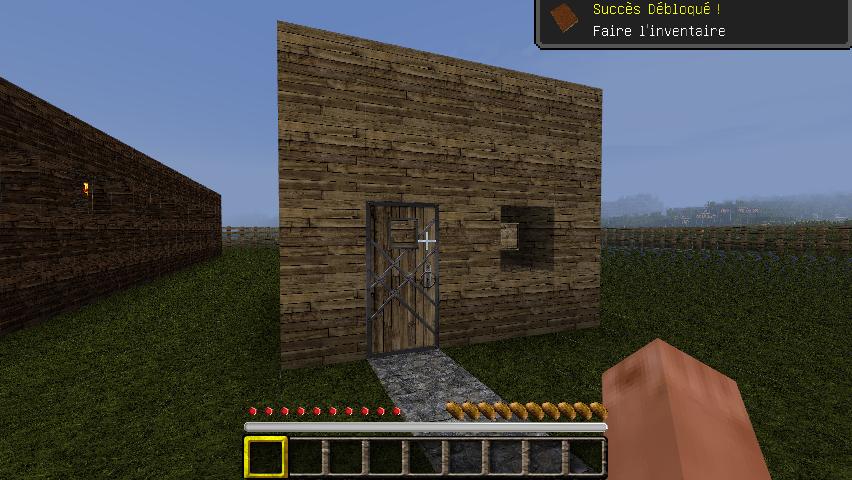The image portrays a Minecraft scene with a central focus on a wooden structure. The structure features wooden tiles resembling a wall and a door with cross-like designs on its right side. Adjacent to the door is a square section, possibly indicative of a window, and an actual window to its immediate right. The ground is primarily green, punctuated by a gray walkway. To the left of the structure, there's a large brown block. The background sky is blue with a hazy, foggy appearance. In the distance to the right, fencing is visible. At the top right corner of the screen, French words "success, développeur, inventeur" are displayed, indicating achievement messages. The player's interface shows hands extended, full health, full food bars, and an empty inventory grid.